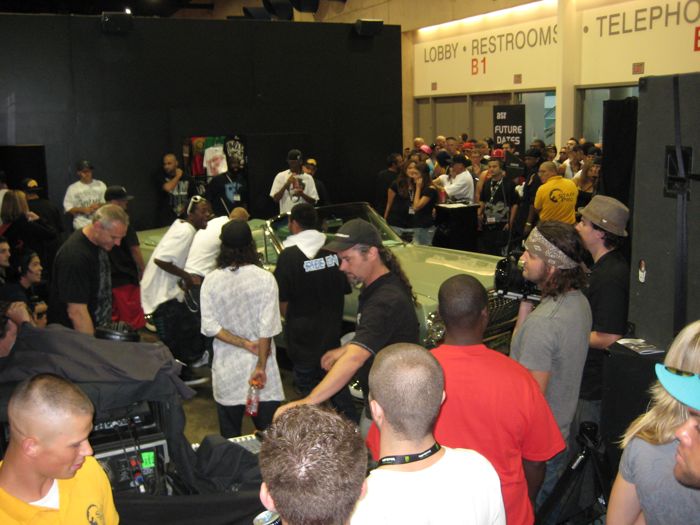The photograph captures a bustling scene at what appears to be an indoor car show or exhibition held in a convention center. The backdrop features signs indicating "Lobby," "Restrooms," "B1," and "Telephone," suggesting a large, organized venue. An eye-catching lime green, 1950s-style convertible is prominently displayed, drawing a crowd of mixed attendees who are gathered closely around it. The crowd is diverse, composed of people of various races and ages, dressed in an array of styles. Among the observers, there are individuals equipped with video cameras and electronic gear, hinting at possible media coverage or a DJ setup. Temporary black walls contrast with the convention center's expansive white walls, creating a structured, yet temporary environment filled with the excitement of the event. The scene blends the enthusiasm of car enthusiasts with the professionalism of media personnel, making it a vibrant, energetic snapshot of the exhibition.